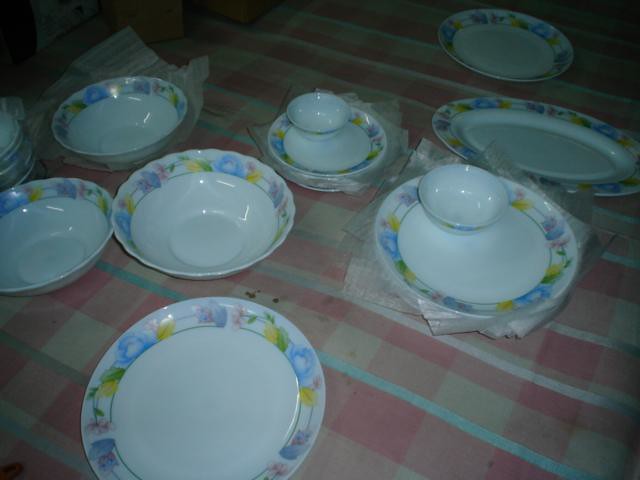This poorly lit, indoor photograph showcases a collection of white china dishes meticulously arranged on a pink, blue, white, and beige checkered tablecloth. The dishes, adorned with a delicate floral pattern featuring blue, yellow, and pink flowers with green leaves, include two plates, each with a matching bowl, three small bowls likely used for soup such as miso, and one saucer paired with a teacup. An elongated oval-shaped platter can be seen in the background. The overall lighting is dim, casting shadows and causing reflections on the shiny surfaces of the china, with darker areas suggesting a distant light source. Additionally, some translucent paper is placed underneath and between certain dishes, perhaps for protective purposes.